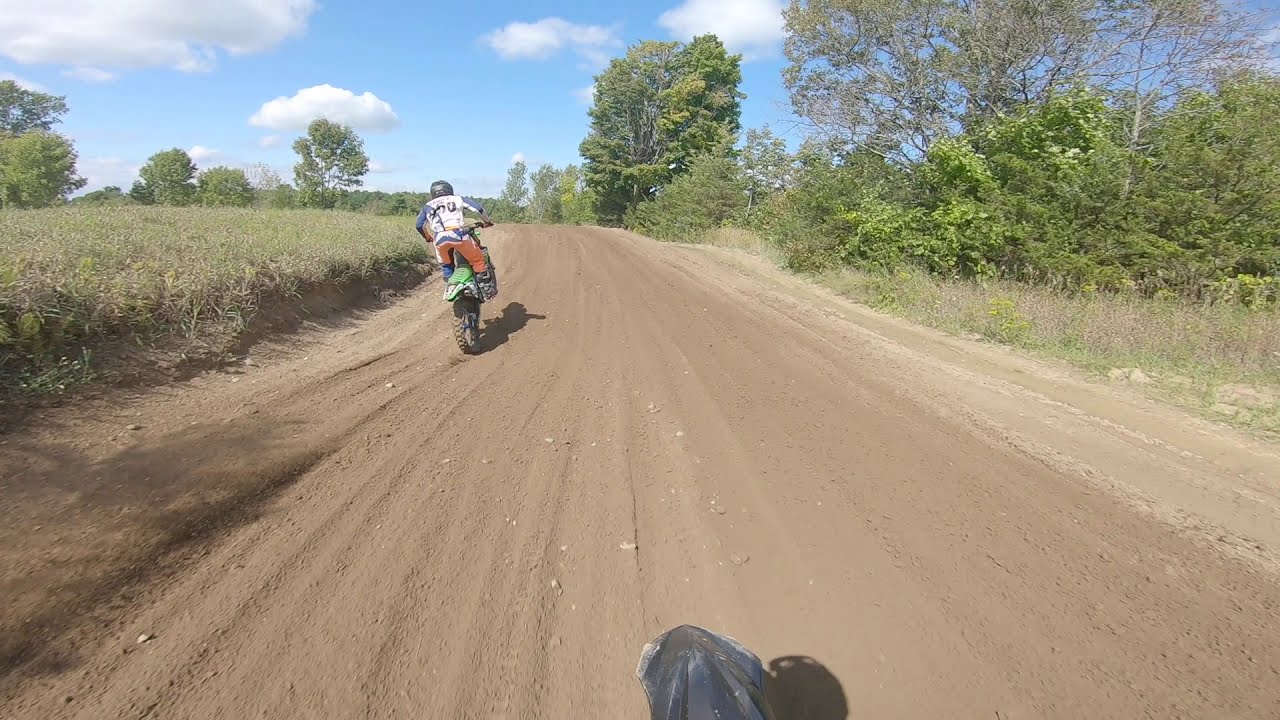This point of view photograph captures the thrilling experience of riding a dirt bike on a well-traveled dirt road. The road itself is composed of soft brown dirt marked with multiple tire tracks, indicating its frequent use. In the lower part of the image, only the black front tire of the narrator's dirt bike is visible. Ahead on the road, another rider on a yellow and white dirt bike, which sports brown and black tires, captures the eye. This rider is wearing distinctive orange pants, a white jacket, and a black helmet. The road is bordered by green and tan vegetation, extending to dried grass and shrubbery. In the distance, multiple trees with lush green leaves stand under a wide expanse of blue sky dotted with sporadic white clouds. The scene conveys a sense of adventure and open-air freedom, set against a picturesque natural backdrop.